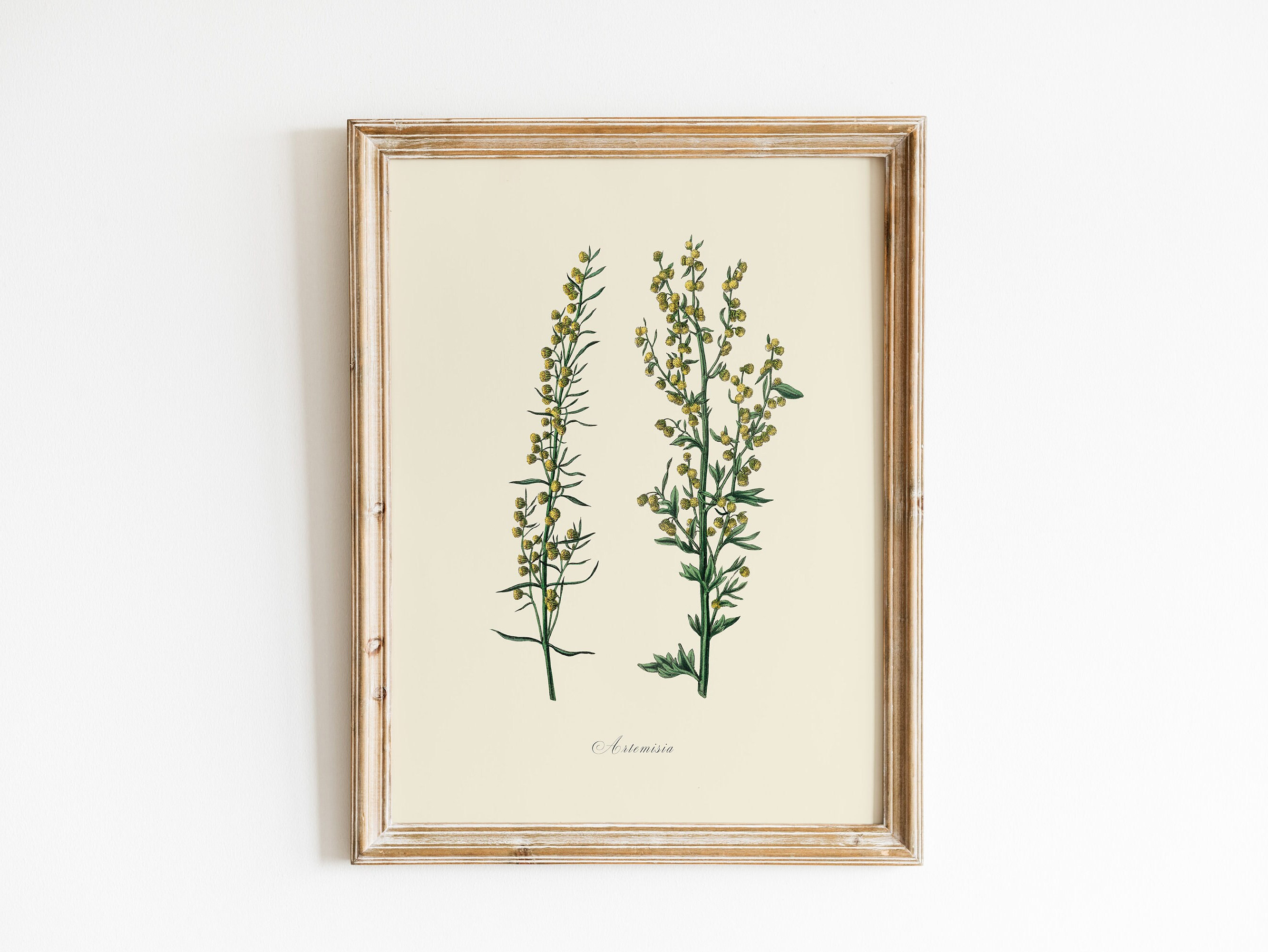This photo features a framed image, which appears to be a painting or computer-generated picture, hanging on a white wall. The frame is an elegant birch wood with a rustic tan finish, complementing a beige background within the artwork. The focal point of the image showcases two green plants with numerous slender sprigs. The left plant is characterized by a single, more slender twig, while the right plant is slightly robust with a few small branches. Both plants are adorned with small yellow buds, some described as pom-pom flowers or yellow balls. Underneath these plants, a small word in cursive is inscribed, spelling "A-I-T-E-M-I-S-I-A," which is potentially the name of the plants or the artist's signature.